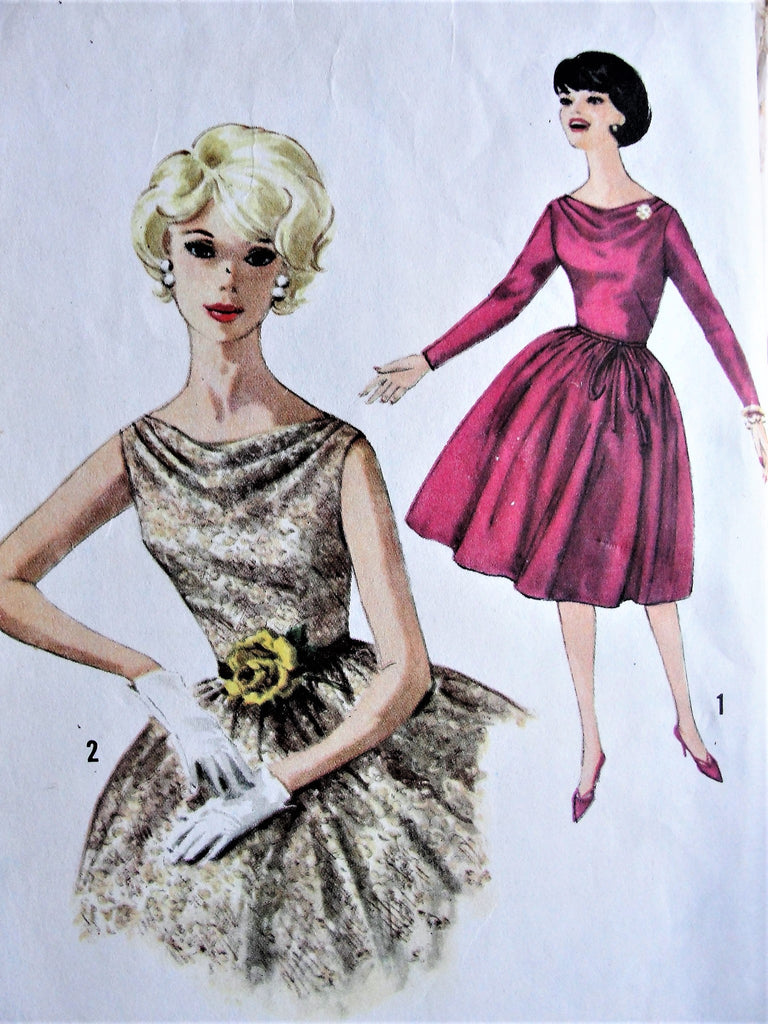The image is a vintage fashion illustration featuring two women dressed in mid-20th century attire, likely from the 1950s or 1960s. The woman in the foreground, positioned on the left side, has short blonde hair and is smiling gently. She is adorned with pearl earrings and white gloves, and her dress is a shimmering golden color with a gray floral pattern, cinched at the waist with a black belt featuring a prominent yellow flower. The second woman, illustrated in the background on the right, has short dark hair and poses with her hands slightly outstretched as if in mid-dance. She wears a purple dress with long sleeves and a purple rope belt, accented by a little jewelry brooch on her left shoulder. Her outfit is complemented by matching purple heels. Both illustrations exude a vintage charm, reminiscent of fashion magazine pages or dress patterns from a bygone era, designed to inspire women to create their own stylish dresses.